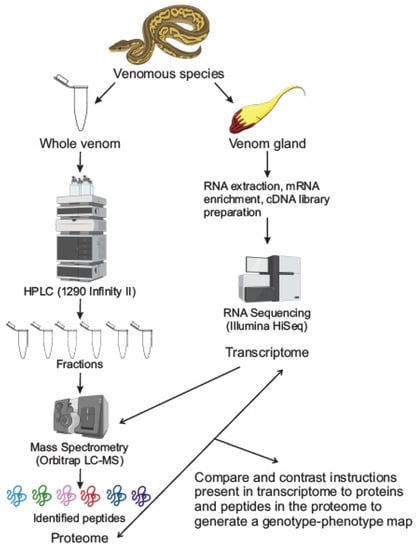The image is a detailed flowchart from scientific literature, showcasing the processes involved in the analysis of snake venom. 

At the top center, a snake labeled "Venomous Species" serves as the starting point. From here, the flowchart splits into two main paths: the left side focuses on whole venom analysis, while the right side emphasizes RNA extraction from the venom gland.

On the left path, below the snake, a test tube labeled "Whole Venom" is depicted. An arrow points to an "HPLC 1290 Infinity 2" machine, followed by more test tubes labeled "Fractions." A subsequent arrow leads to a "Mass Spectrometry, Orbitrap LC-MS" machine. Further down, another arrow points to "Identified Peptides," represented by colorful squiggles.

On the right path, an organic-looking structure labeled "Venom Gland" leads to the text "RNA Extraction, mRNA Enrichment, cDNA Library Preparation." An arrow from here points to an "RNA Sequencing, Illumina HiSeq" machine. This then connects to the term "Transcriptome."

At the bottom, both paths converge with arrows pointing to a comparative section between "Identified Peptides" and "Transcriptome," labeled "Proteome." This illustrates the integration of proteomic and transcriptomic data to generate a more comprehensive understanding of the venom’s properties.

The entire flowchart is visually enriched with illustrations of scientific equipment and process steps, making it a thorough depiction of the intricate methods used in venom analysis.